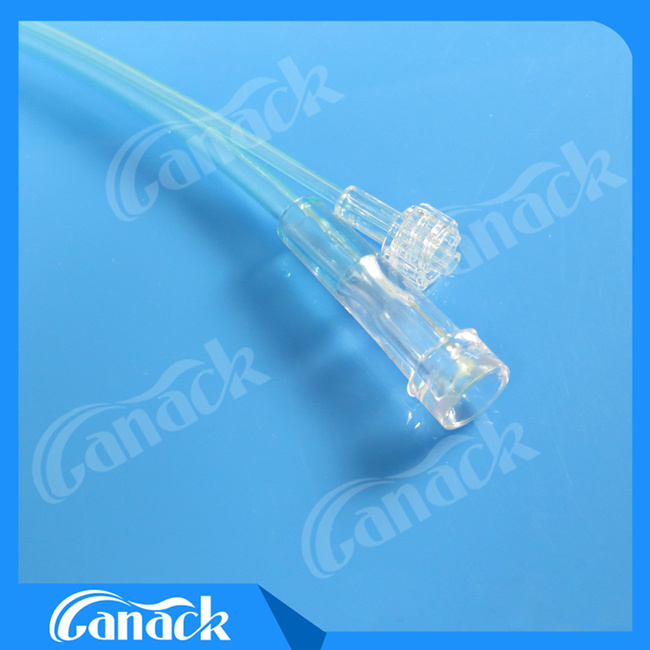The image displays a pair of clear plastic tubes, possibly medical devices such as catheters or IV lines, set against a well-lit, light blue background with a slightly darker blue rectangular border. The tubes, one slightly longer and wider than the other, originate from the upper left corner and sweep towards the lower right, causing shadows to cast towards the bottom left. The image includes several watermarks of the brand name, which resembles "Canack" or "Ganack" (C-A-N-A-C-K or G-A-N-A-C-K) written in a proprietary, wavy cursive-like font. These watermarks appear four times around the tubing—above, below, left, and right of the tubes. Additionally, the same branded text is prominently featured in the bottom left corner of the blue border, with a small dark blue prism on the right side of this corner, giving an illusion of a folded down section. The exact scale and specific details of the tube endings are uncertain.